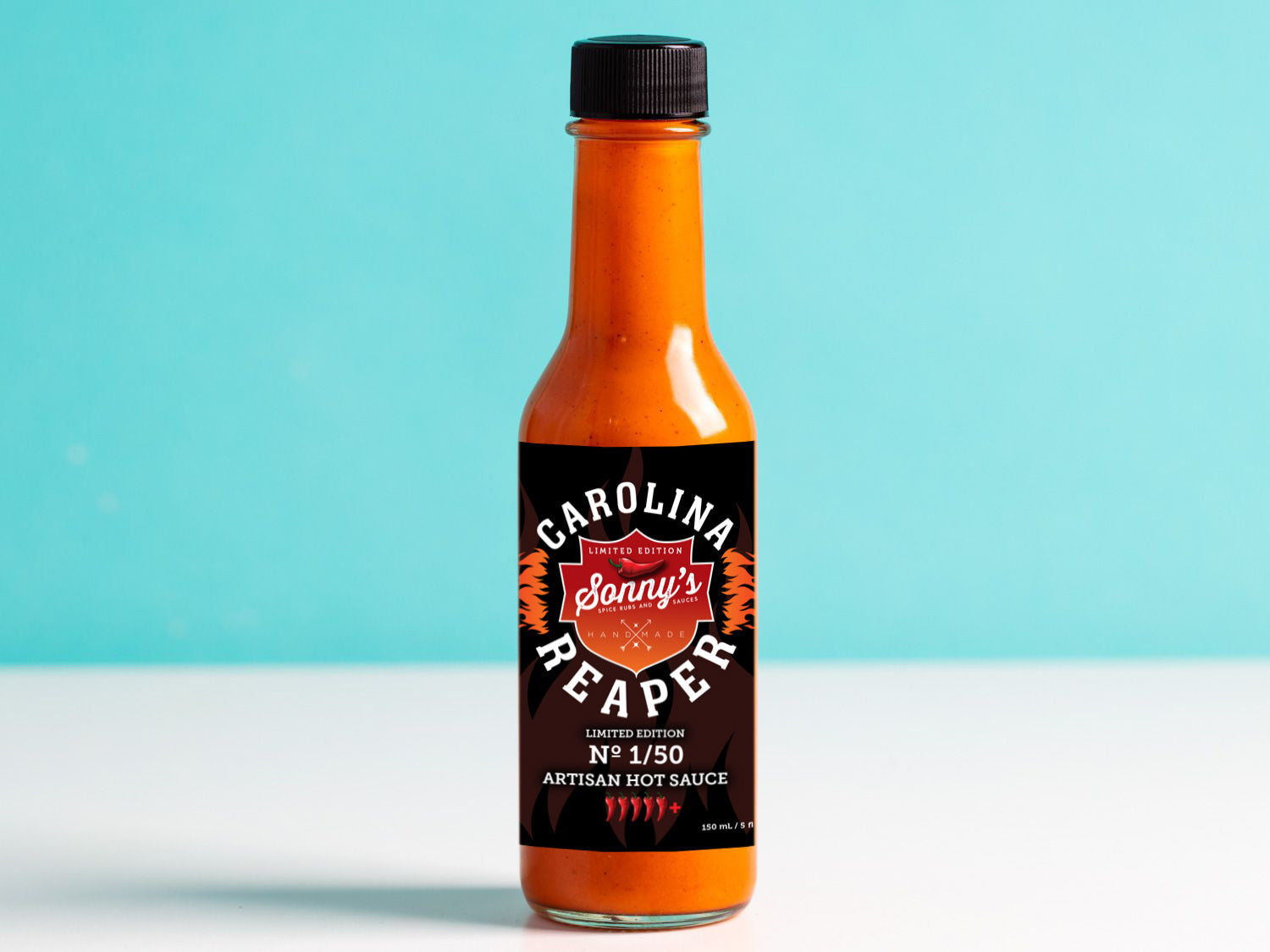In this vibrant advertisement, a bottle of limited edition Sonny's Carolina Reaper hot sauce takes center stage against a bright blue background. The bottle, crafted from glass, stands on a blurry white surface, casting a shadow to the left. It features a wide bottom that slightly narrows towards the top, capped with a black, rigid plastic top.

The bottle's label is predominantly black, adorned with a reddish-orange shield. At the top of the shield, a red chili pepper is depicted, followed by the word “Sunnies” in elegant white script. Flanking the shield, in bold white capital letters, is the text "Carolina Reaper." Below this, meticulous white text reads "Limited Edition," highlighting the product's exclusivity.

Handmade and artisan-style, this hot sauce boasts a hefty 150 milliliters (5 fluid ounces) of spicy Carolina Reaper goodness. The label also indicates a small batch production number, marked as 1-50, emphasizing its rarity and premium quality. Designed to add a fiery kick to any dish, this small-batch hot sauce promises an extraordinary culinary experience.